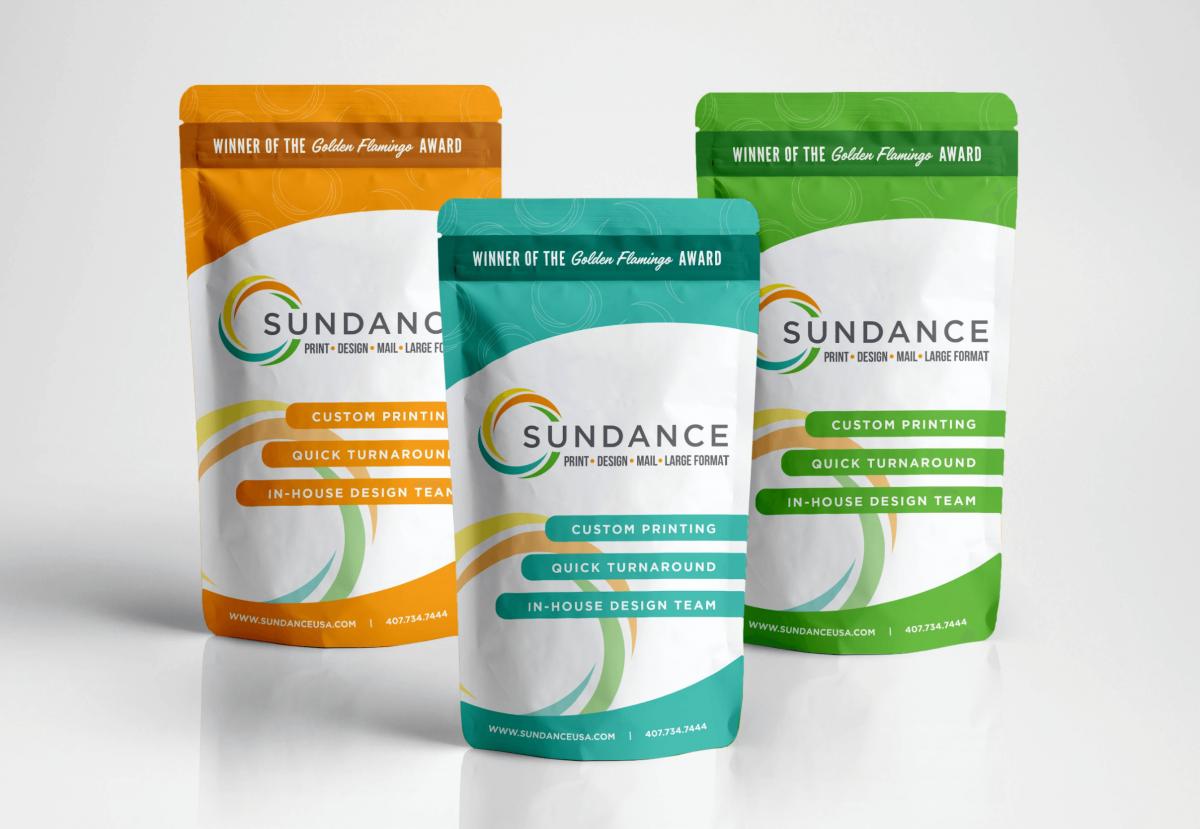This landscape-oriented color photograph features three vertically arranged product pouches displayed against a light gray background, reminiscent of a stock image used for commercial purposes. Each pouch prominently showcases the text "Winner of the Golden Flamingo Award" across the top. Below this, the brand name "Sundance" is printed in black lettering next to a twisted color circle with bands of orange, red, green, and blue. The elliptical white section on the front of each pouch contains the text "Print, Design, Mail, Large Format," followed by company attributes highlighted in horizontal strips: "Custom Printing," "Quick Turnaround," and "In-House Design Team." At the bottom, the pouches provide the contact information "www.SundanceUSA.com" alongside a phone number.

The pouches differ only in color: the one on the left is an orange-yellow, the middle one is aqua blue with white accents, and the one on the right is grass green. Notably, the aqua blue pouch is positioned slightly forward and angled towards the viewer, adding depth to the composition. The overall style of the image is photographic realism, emphasizing clear and precise details for marketing purposes.